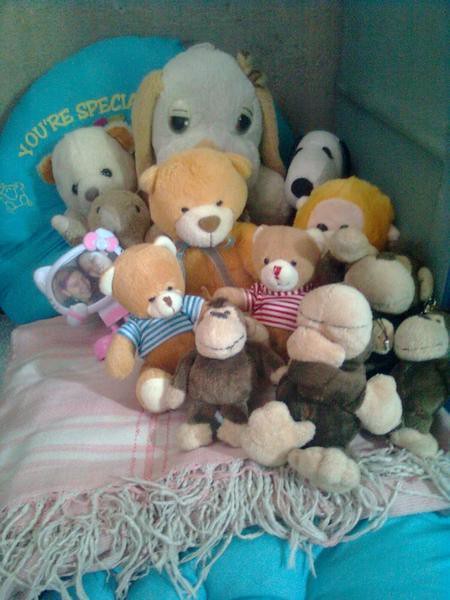This image showcases a cozy corner, likely part of a bedroom, featuring a cluster of stuffed animals on a bed. The bed has a light sky blue or cyan cushion, topped with a folded pink and white plaid blanket adorned with white frills. Arranged on this blanket is a collection of eleven stuffed animals, including four monkeys with large stuffed faces and short fur, three teddy bears, a panda, and a few indistinguishable plush toys. Prominently, there's a large gray dog with half-lidded eyes and a Snoopy stuffed animal. Adding a personal touch, a pillow in the background reads "You are special," and nestled among the plushies is a picture frame shaped like Hello Kitty containing an image of two people with hearts around them. The animals are neatly positioned to face the camera, creating a heartwarming and intimate scene.